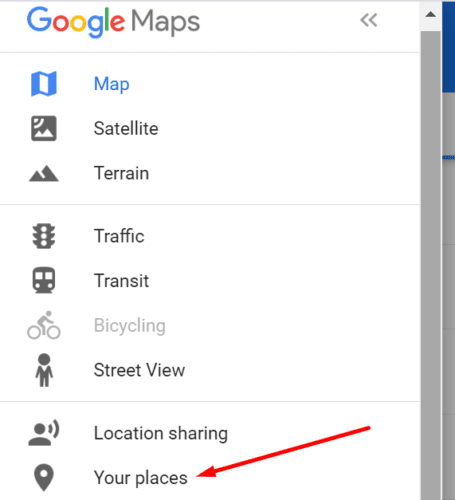This image showcases the settings menu for Google Maps in meticulous detail. At the top of the interface, the iconic Google logo is prominently displayed in vibrant, multicolored letters: the 'G' is blue, the first 'O' is red, the second 'O' is yellow, the second 'G' is blue, the 'L' is green, and the 'E' is red. The word "Maps" is written in a subtle gray color directly below the logo. 

Beneath the logo is a thin gray line that separates the branding from the menu options. The menu is organized into two distinct columns: one for icons and one for text descriptions. The first icon is a blue map symbol accompanied by the word "Map." 

Following this, the text list reads in order from top to bottom: "Satellite," "Terrain," "Traffic," "Transit," "Bicycling," "Street View," "Location Sharing," and "Your Places." Each of these text labels corresponds to an icon in the adjacent column. The icons, in order from top to bottom, are: a satellite symbol for "Satellite," a mountain symbol for "Terrain," a stoplight for "Traffic," a bus for "Transit," a bicycle for "Bicycling," and a person for "Street View." 

Significantly, a long, thin, red arrow is pointed directly at the "Your Places" text option, drawing special attention to this section of the menu.